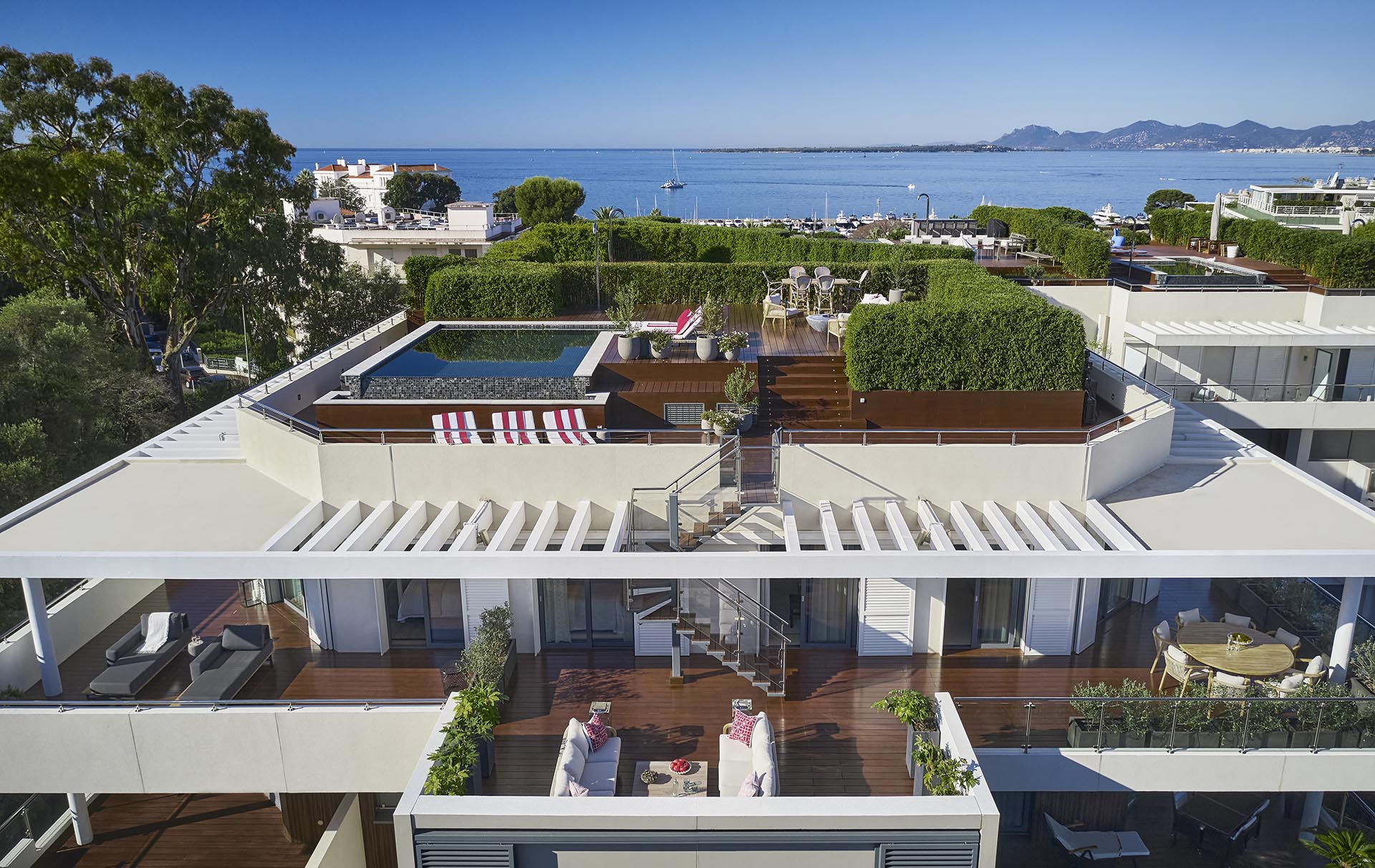This aerial photograph captures a modern, multi-level white mansion overlooking a vast expanse of water, bordered by hills and mountains on the right. The rooftop level features a clear blue swimming pool surrounded by a wooden deck with three striped canvas lounge chairs, white and red, and a maze-like arrangement of tall green hedges. There is a set of wooden steps leading to a rooftop area adorned with a round table and several chairs for sunbathing. The level below showcases various seating arrangements, including a set of white loveseats with a coffee table in between, flanked by pink pillars. Also, there's a round table with eight white cushioned chairs and an expansive outdoor dining area. Along the wooden flooring, multiple sliding glass doors open onto this deck, suggesting it could be a hotel or an exceptionally large house. The lower deck extends with more seating areas and lounge chairs on the left. In the background, several smaller white buildings and boats moored near the shore add to the picturesque setting.